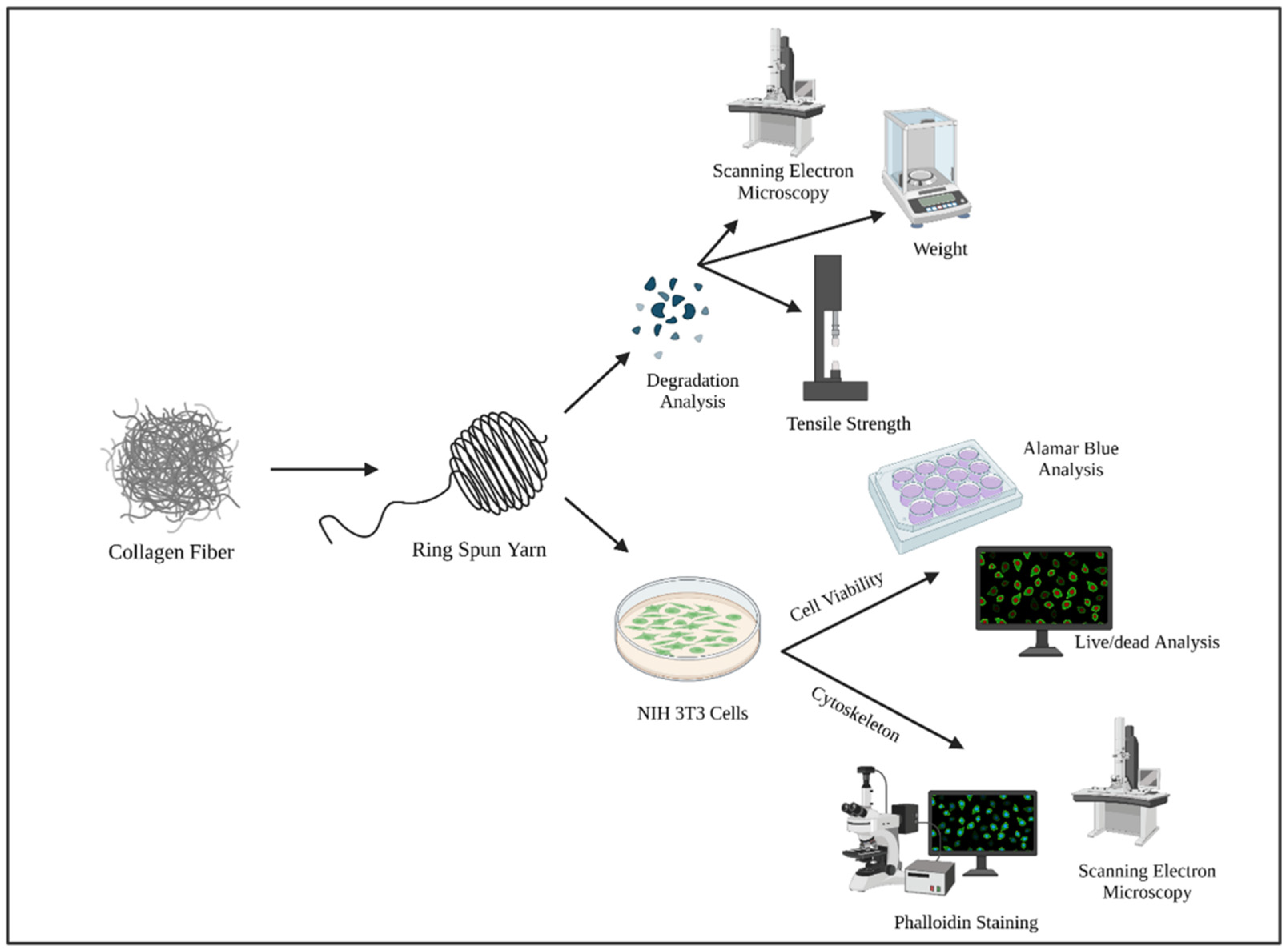This colored illustration, combining intricate drawings and informative typography, is a detailed flowchart explaining the in vitro biocompatibility and degradation processes of polymers. The landscape-oriented image, set against a white background framed by a thin black rule, is replete with small images and annotations concentrated on the right side, gradually tapering towards a central illustration on the left.

At the top right, the flowchart starts with a drawing of a microscope labeled "Scanning Electron Microscopy," showing an individual performing the task. Just below, another image depicts a laboratory scale with the label "Weight." Beneath it, an arrow points to a columnar device marked "Tensile Strength." To the left of this machine is a cluster of purple ovals labeled "Degradation Analysis."

Continuing downward on the right, the next illustration features a computer monitor displaying green circular areas on a black background, representing "Live/Dead Analysis." Further down are two microscopes and another computer screen, indicating additional scientific procedures. Below these, another monitor and labeling highlight areas of "Cell Viability" and "Cytoskeleton." 

On the left side of the image, central illustrations depict a ball of yarn, initially labeled "Collagen Fiber," which transitions into "Ring Spun Yarn." From the yarn, arrows extend upwards to the aforementioned degradation analysis and SEM images, and downwards to a pink container, suggesting a petri dish, with green specks, labeled "Alamar Blue Analysis."

Overall, this technical flowchart uses arrows and detailed annotations to guide the viewer through a comprehensive visualization of scientific analyses, capturing the complex interplay between various testing instruments and the related polymer degradation processes.